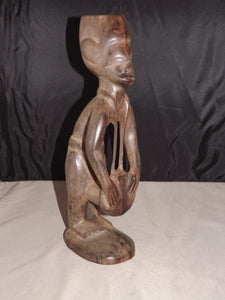The vertically aligned rectangular image depicts an ancient-looking sculpture that might have been unearthed from an archaeological dig, suggesting it could be hundreds or thousands of years old. Placed on a white marbled surface table with beige and gray undertones, the statue stands against a black, silky, and wrinkled background that resembles a curtain or sheet. The sculpture, which seems to be carved out of wood, features natural brown tones with lighter brown and white accents. Approximately two feet in height, the figure, which might represent a man or a native Indian, showcases a flat-topped head with ears carved out. Its face lacks detailed features, adding an archaic charm. The arms hang down, holding what appears to be a satchel with intricately carved straps extending up to the shoulders. Dressed in a half sarong that hangs from its waist, the figure's feet are joined together and rest on a round wooden base. Despite the professional lighting, there is a slight softness to the focus, which does not detract from appreciating this carefully carved, perhaps spiritual or cultural, figurine.